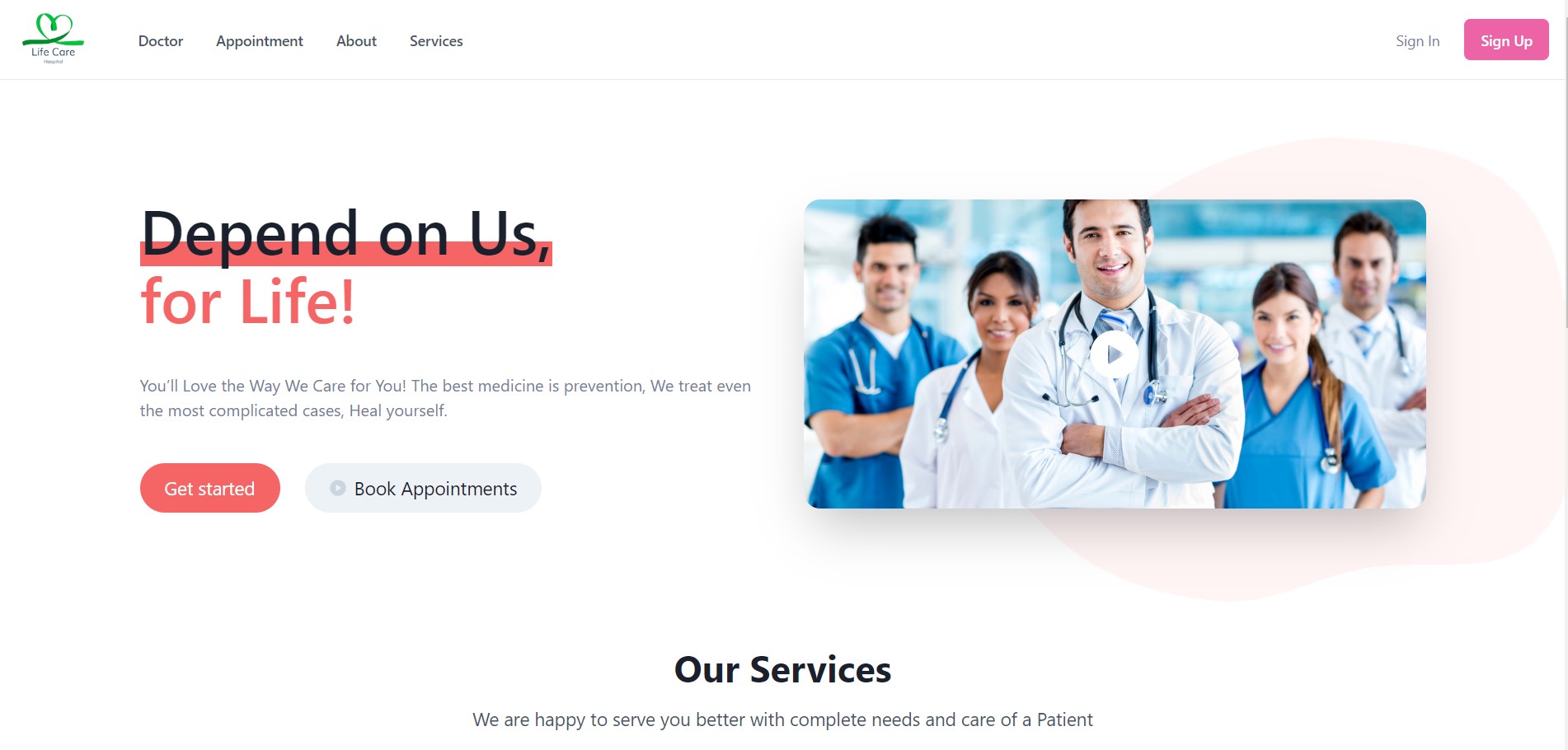This screenshot from a website features a white background with a square image prominently displayed, showcasing five medical professionals. From left to right, the professionals are as follows:

1. A man with dark hair dressed in a blue tunic.
2. A woman of Asian descent, attired in a white tunic with a stethoscope draped around her neck.
3. A white man with dark hair, also wearing a white tunic and a stethoscope.
4. A woman with long dark hair, clad in a blue tunic.
5. Another man with long dark hair, dressed in a white tunic and featuring a stethoscope around his neck.

To the left of this image, a vibrant red banner highlights the words “Depend on Us.” Beneath this banner, the slogan continues in red text: “For Life.” The message underneath reads in smaller text: "You'll love the way we care for you. The best medicine is prevention. We treat even the most complicated cases. Heal yourself."

Below this message, there are two pill-shaped buttons for user interaction:
- A red button with the text "Get Started"
- A gray button reading "Book Appointments"

At the very bottom, the text highlights the website's services: "Our Services: We are happy to serve you better with the complete needs and care of a patient."